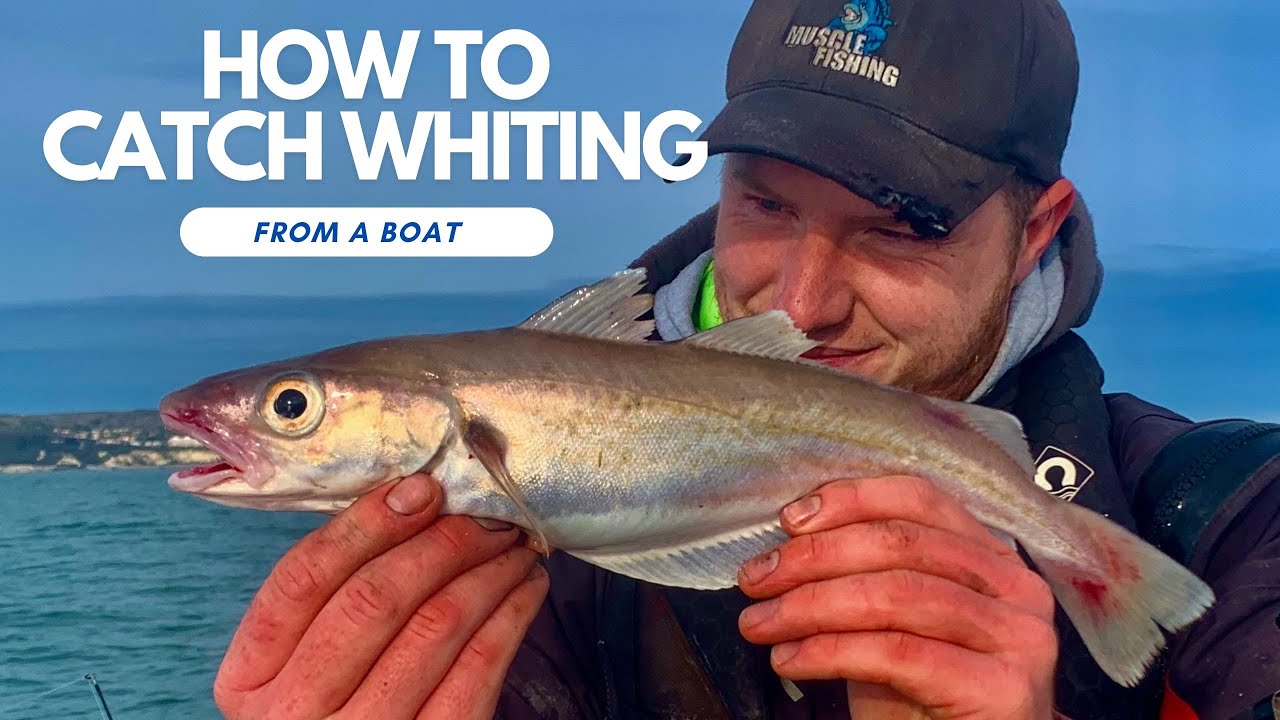The image appears to be the cover of a book or a video thumbnail titled "How to Catch Whiting from a Boat." The photograph prominently features a white man with a thin beard and a mustache, set against the backdrop of open water with a small strip of land in the distance. He is holding up a long, shiny whiting fish with both hands, which are noticeably bright red, likely from the cold. The fish, positioned towards the left side of the image, has an open mouth and a large eye, with slight red discoloration around its mouth and tail. The man is squinting and admiring the fish, analyzing it up and down, while facing the camera at an angle.

He is wearing a dark-colored coat over a gray hoodie and a neon yellow hoodie, topped with a baseball hat that bears the logo "Mussel Fishing" and appears tattered at the brim. The text "How to Catch Whiting" is in white in the upper left corner, with the phrase "from a boat" in blue within a large white oval below it. The sky is bright blue, occupying a significant portion of the background, and the ocean appears blue and choppy, emphasizing the outdoor, maritime setting.